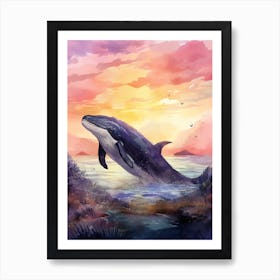The image depicts a detailed artwork in a vertically oriented, black rectangular frame with a white inner border, set against a white wall. The central focus of the artwork is a majestic killer whale, distinguished by its iconic black and white coloring, leaping out of crystal blue water. The whale is captured in mid-air, angled towards the left with its tail down and to the right. Surrounding the whale, the vibrant sky showcases a breathtaking gradient of colors—light blue, pink, white, gray, red, and orange—suggesting either a sunrise or sunset, complete with scattered clouds. In the foreground, there is a brown and green landmass sweeping across the image, complemented by a puddle of water at the very front. The artist has masterfully blended elements of nature, including plants at the bottom right and left of the artwork, making use of watercolors to bring this serene and dynamic scene to life.